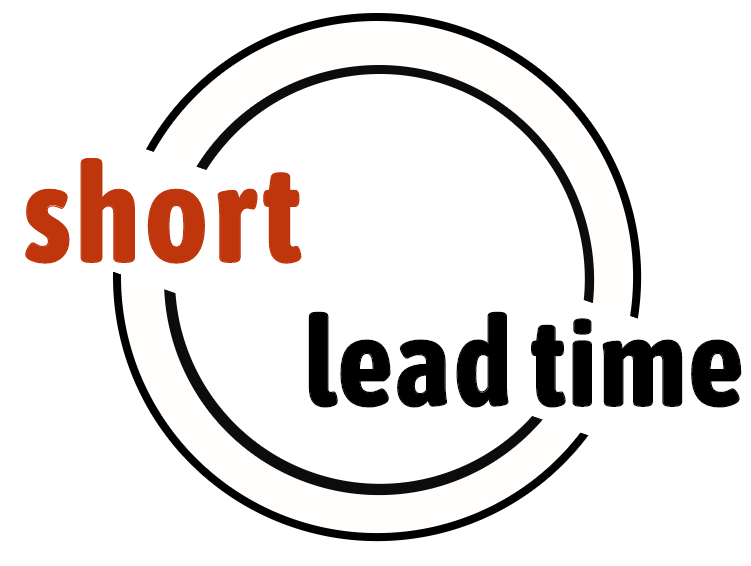The image features a clean, minimalist design that has a dual-circle motif, with an outer and an inner circle. Both circles are interrupted by the text they contain. On the upper-left side of the image, the word "short" is displayed in a large, dark red (burnt orange) lowercase font. Below and to the right, the phrase "lead time" appears in the same font style but in black. The words "short" and "lead time" break the continuity of the circles, making the letters pop out distinctly. The background within the circles is white, emphasizing the text. This visually striking design seems tailored for an advertisement, delivering a clear and concise message about a short lead time in a highly eye-catching manner.